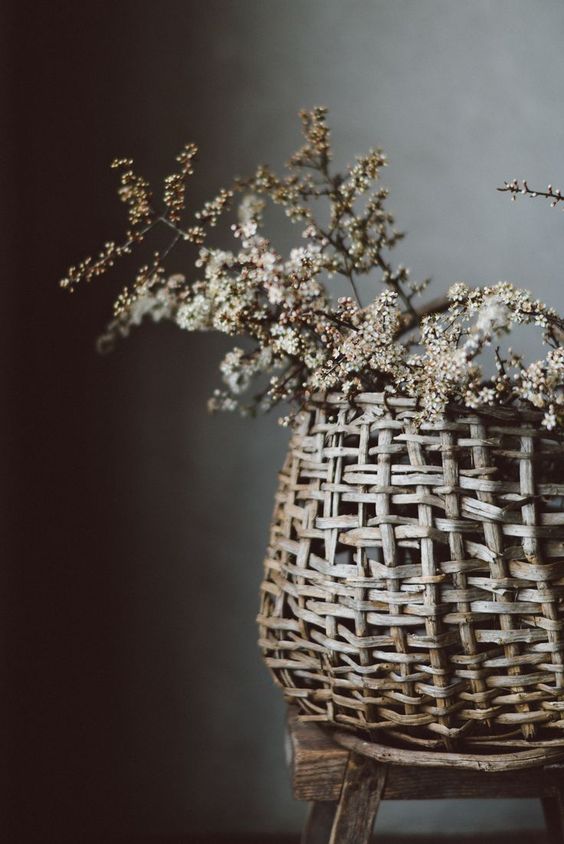In this color photograph, the background transitions from a pitch black on the left to a smoky pale gray on the right. Dominating the right side of the image is a dark brown wooden stool, atop which sits a hand-threaded wicker basket in shades of white and tan. The basket, flush with the center of the photo, contains numerous branches with white flowers. Some of the wicker weaves are broken. The black stems and brown foliage of the branches add depth, with the flowers and plants extending diagonally toward the top left corner. The image is taller than it is wide, devoid of any writing, people, animals, or additional structures.